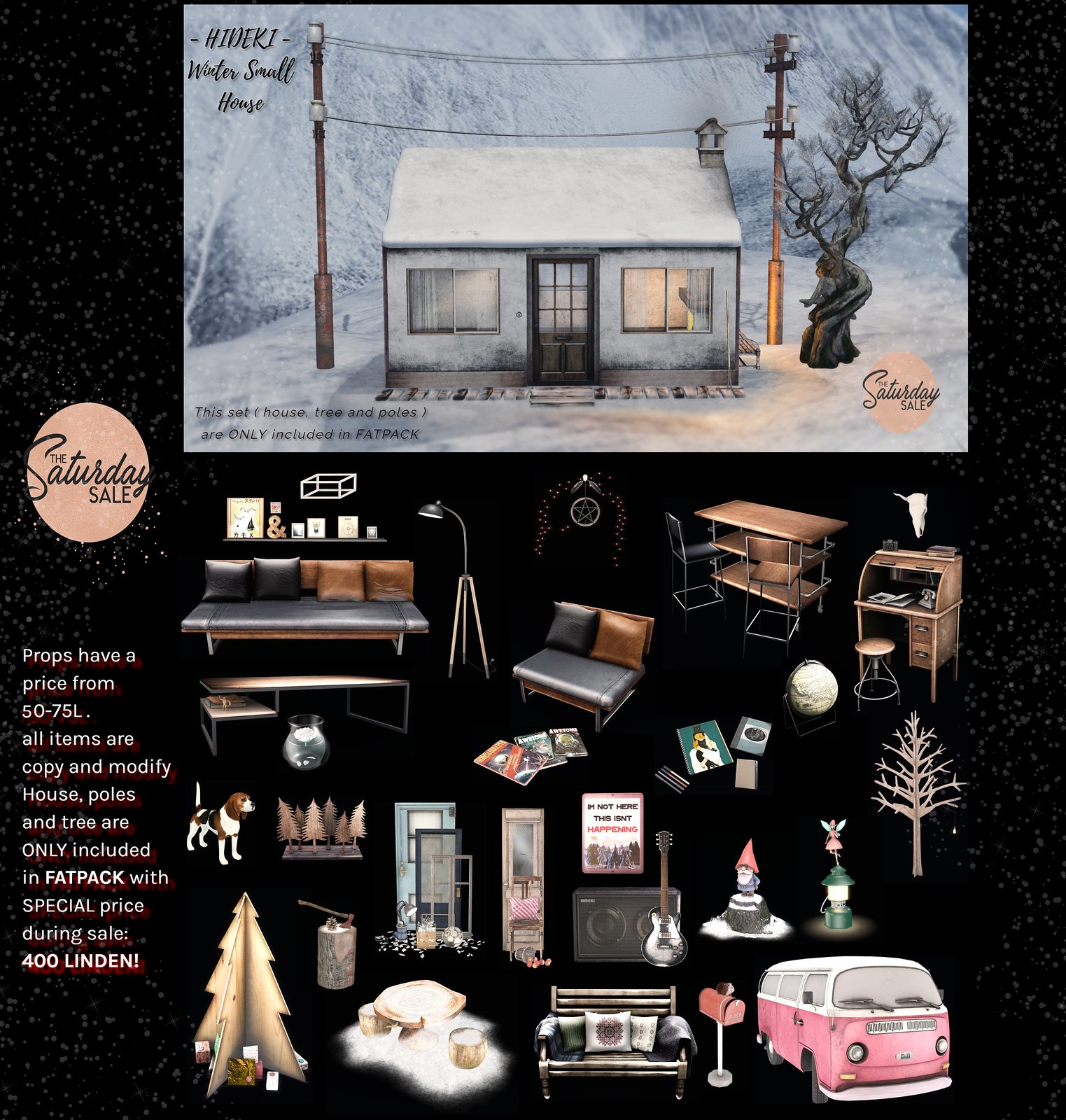The image depicts an intricately detailed miniature model of a small house set against a black background, giving a wintery feel with snow draped over the roof. The house features a front door and two windows, with two telephone poles standing on either side. Illuminated from within, it exudes warmth amidst the cold setting. To the left, the text "The Saturday Sale" is prominently displayed. Below, smaller text clarifies that the set includes the house, tree, and poles, available as a "Fat Pack" for a special price during the sale. Additionally, various miniature props are shown, including a twisted tree, a wooden porch, a bench, a lamp, a guitar with an amp, a wooden Christmas tree, a small desk, tables, a globe, scattered magazines, a hippie van, a mailbox, firewood with an ax, and a beagle. The prices for these props range from 50 to 75 Lindens, and all items are specified as copy and modify. The overall scene exudes a quaint, picturesque charm, reminiscent of a cozy winter's day.